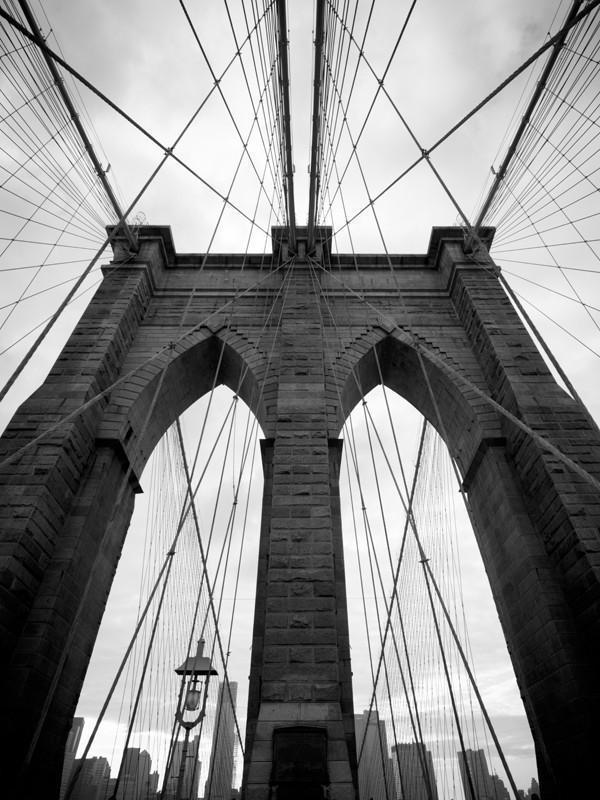This black and white photograph features a towering bridge, likely the iconic Brooklyn Bridge in New York City, captured from a low angle looking straight up. The bridge, constructed from large rectangular stones or bricks, showcases its impressive structural elements, including three tall pylons and two archways. Numerous cables extend from the bridge’s framework, some forming an X-shape, while others fan out to provide stability and support. A high fence lines the perimeter of the bridge, which along with the cables, ensures safety. An old-fashioned streetlight with a pillar and a light fixture is visible in the left archway. In the background, amidst a cloudy gray sky, the distinctive New York City skyline with its towering skyscrapers sets a remarkable scene.